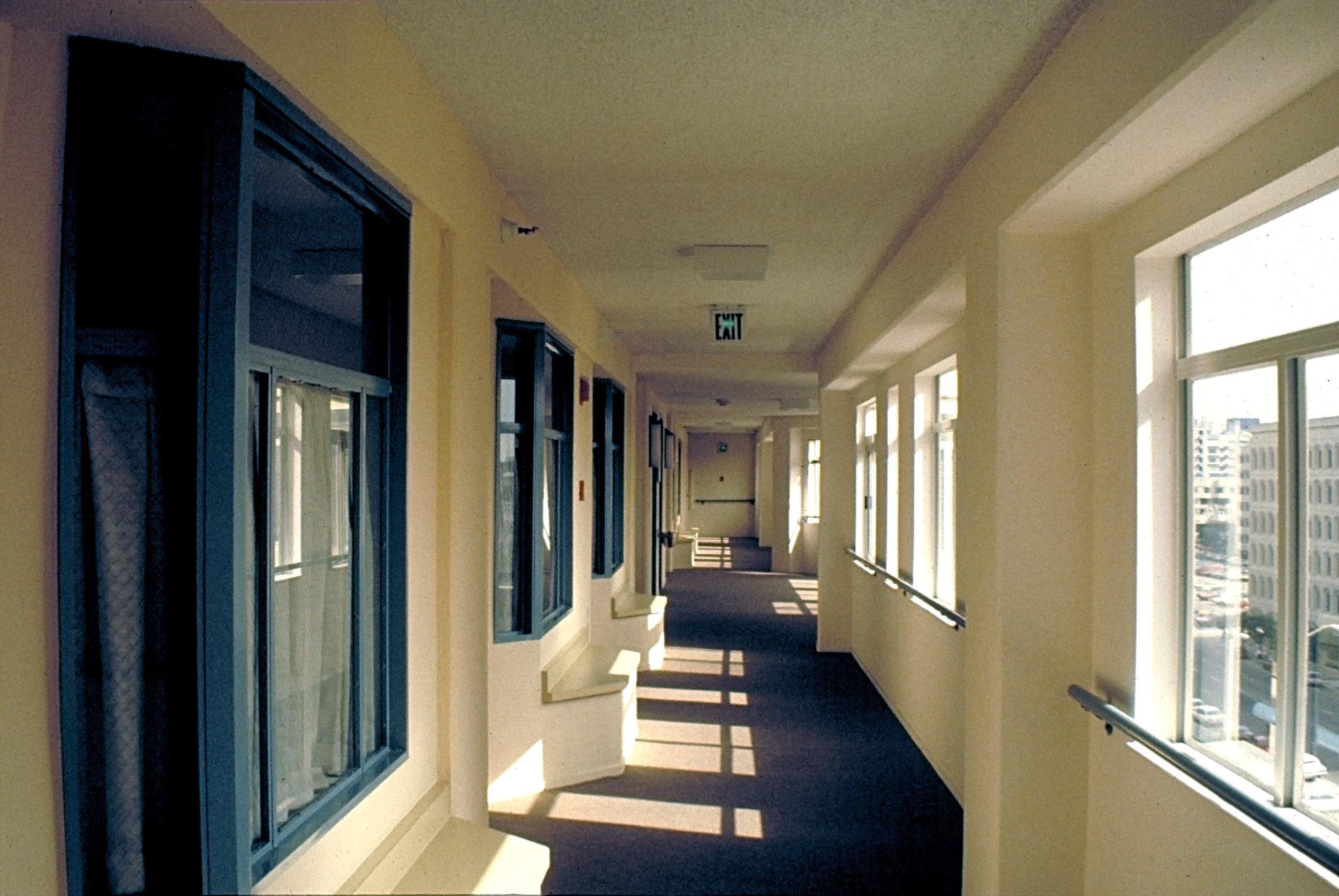The image captures a bright, sunny hallway with white walls and ceiling, and beige carpeting. Sunlight pours through multiple large windows on the right side, creating shadows on the floor and revealing an exterior view of buildings and a seascape under a clear, bright sky. The left side of the hallway features blue-trimmed interior windows with white curtains, likely leading to apartments, each accompanied by a small bench for seating. At the end of the hallway, there is an emergency exit door, and an illuminated green exit sign hangs from the ceiling. Far down the hall, there appears to be a possible left turn, and black railings are visible against the back wall, adding detail to the overall structured ambiance of the space.